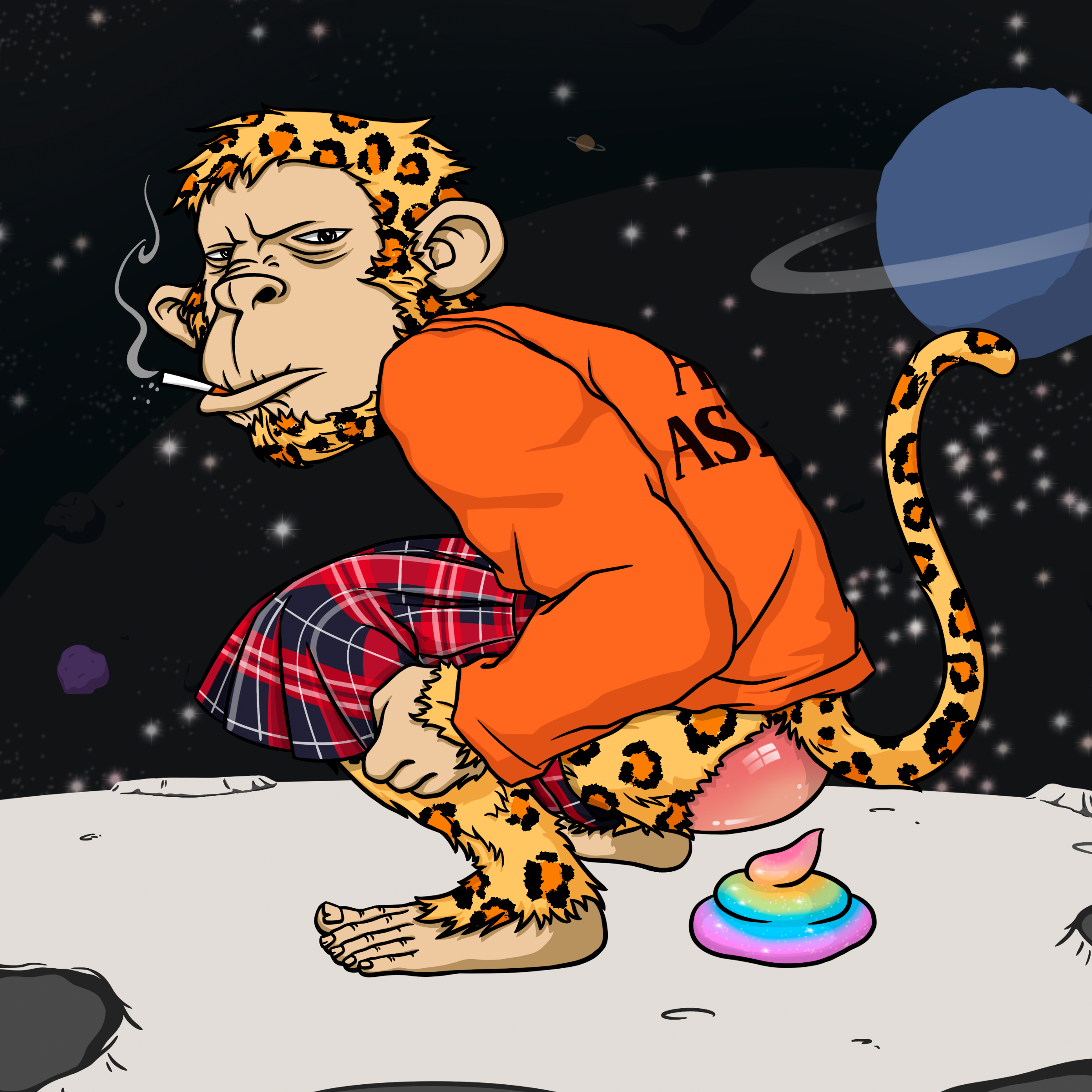The image is an unsettling cartoon depicting a monkey with leopard-like fur, including a cheetah's tail, hair, and beard. This monkey has a cigarette hanging from its mouth, emitting smoke, and is scowling directly at the viewer. It is dressed in an orange prison shirt with partial letters "AS" visible on the back, and a red, black, and white plaid kilt, reminiscent of a Catholic schoolgirl uniform. The monkey is squatting on the lunar surface, pulling down the kilt to reveal its shaved butt as it defecates a rainbow-colored swirl. The backdrop of the scene is outer space, marked by the presence of Saturn in the upper right corner and various stars.